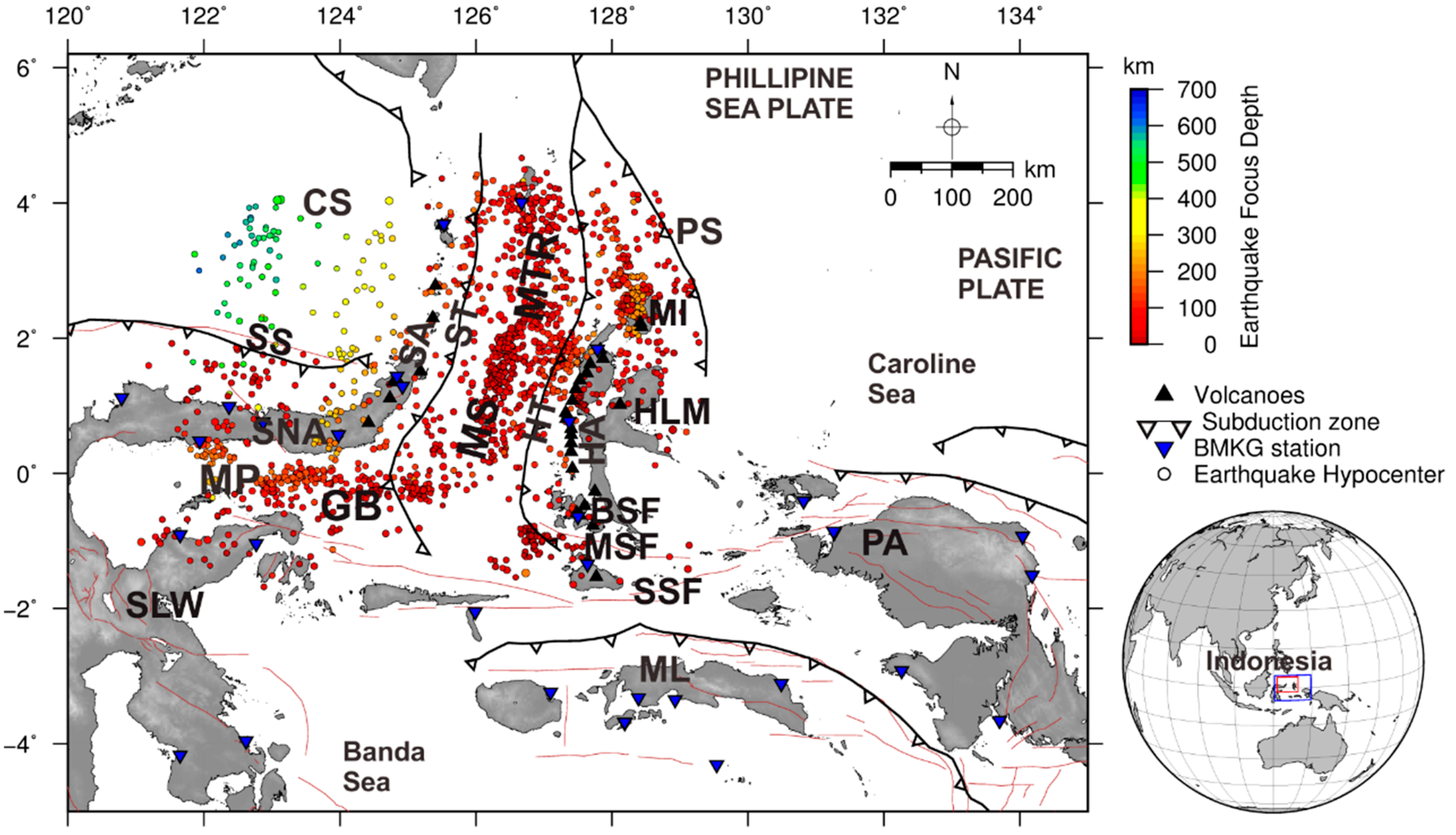This detailed map illustrates seismic activity in the Southeast Asia region, with focus on earthquake focus depth. The map features a color-coded legend on the right, ranging from 700 meters down to zero, with corresponding colors: blue, green, yellow, and red. Additionally, it identifies several key symbols: black triangles for "Volcanoes," inverted white triangles with black trim for "Subduction Zones," a blue inverted triangle for "BMKG Station," and a black-outlined circle filled in white for "Earthquake Hypocenters."

The central image shows a geographic representation of several countries, including Indonesia, as indicated on a globe located in the bottom right corner. Various seas such as the Philippine Sea, Pacific Plate, Caroline Sea, and Banda Sea are labeled throughout the map. The map also includes coordinates along the borders: vertically on the left from -4 to 6, and horizontally at the top from 120 to 134.

Red, green, yellow, and blue dots scatter across the map, indicating different earthquake activities and depths, with labeled areas shaded in gray. The top left highlights labeling systems for observations, including “Philippine Sea Plate” and “Pacific Plate,” reinforcing the map's purpose of depicting seismic and tectonic features. The overall layout is designed to align the geographic and seismic data through its comprehensive legend and labeling, providing insights into the regions’ earthquake dynamics and associated features.